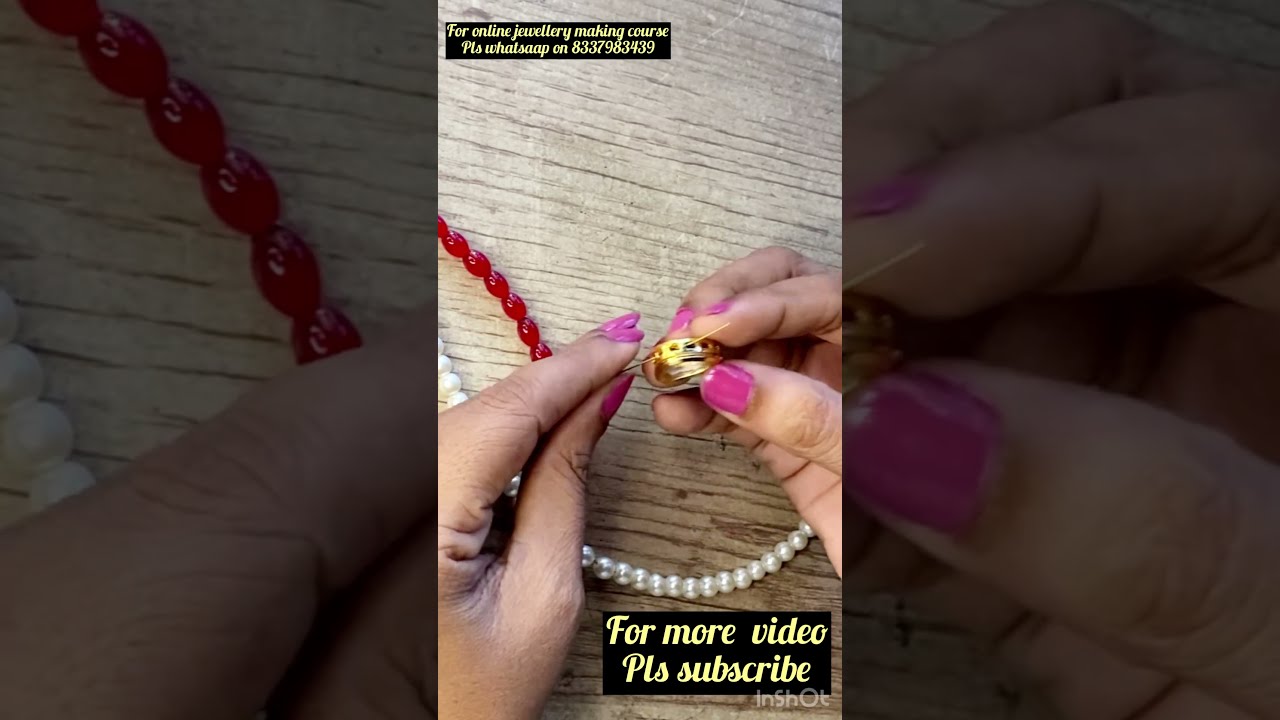In the center of the image is a clear, close-up shot of a woman's hands, distinguished by her pink nail polish. She is carefully threading a needle through a gold piece adorned with holes. Around her hands, on the wooden table, lie an assortment of beads, including red beads and white pearl-like beads. The image is part of a triptych; the larger central picture is flanked by two narrower images on the left and right, showing close-ups of the same jewelry-making process with a darker background, adding depth and focus to the central scene. 

At the top left corner of the image, in a black box with yellow text, it reads "For online jewelry making course, please WhatsApp 833-798-3493." At the bottom center, another black box with white text says, "For more video, PLS subscribe," indicating a call to action for viewers. Additionally, the bottom right corner includes a watermark for the video editing app InShot, hinting that the image was captured from a video, possibly shared on social media. The colors in the image are predominantly brown, pink, gold, red, white, black, and yellow, with the hands and jewelry positioned primarily in the bottom half of the frame.